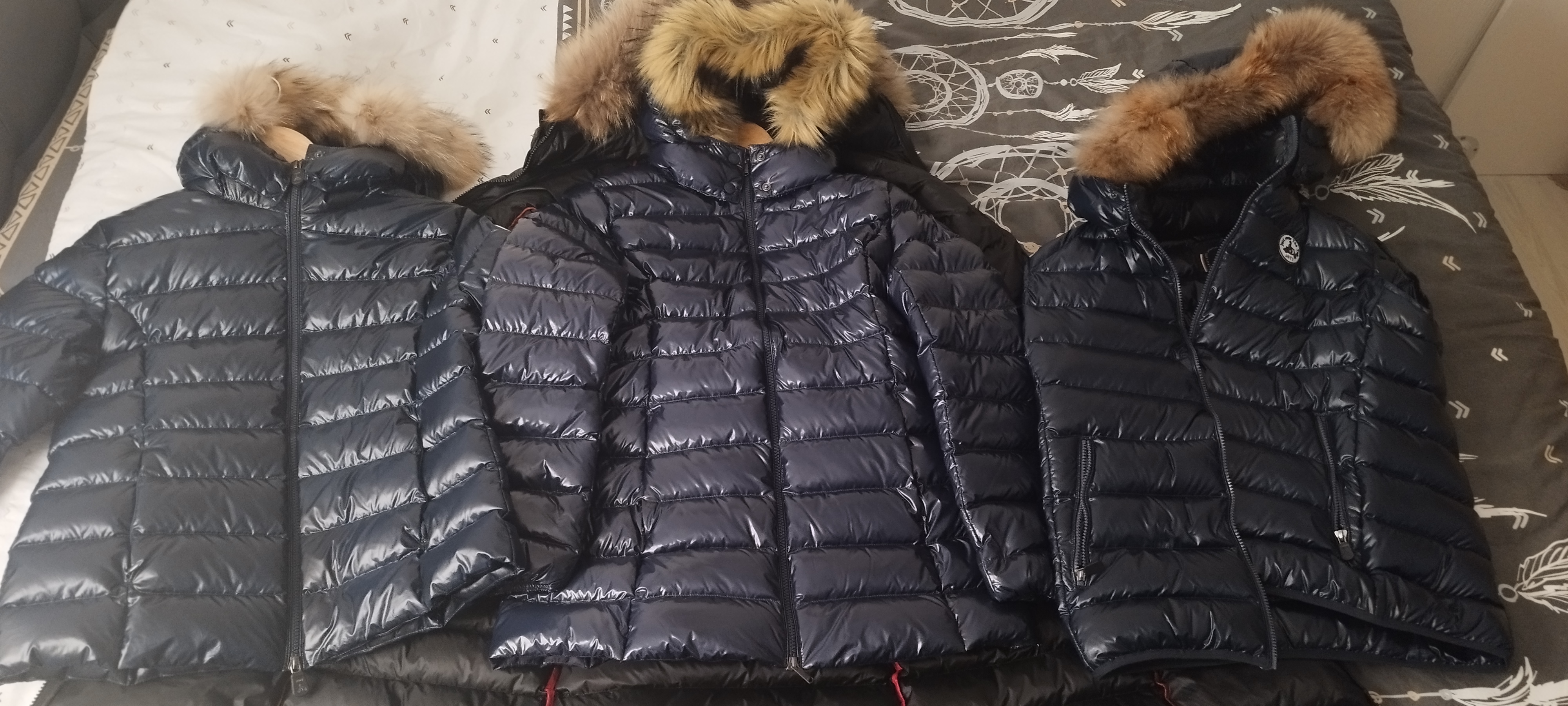This image is an indoor, close-up photograph showcasing a collection of three black women's parka-style puffy jackets, neatly arranged side by side in a single row on a bed. Each jacket is equipped with a zipper down the front and features rectangular puffs and hoods trimmed with thick, light to medium brown faux fur. The jackets vary slightly in size; the leftmost and middle jackets have longer sleeves than the one on the right, which appears sleeker. Notably, the middle jacket seems to be layered atop two other black and gray jackets. The bed beneath them has a cream-colored sheet on the left transitioning to darker brown with a dreamcatcher design on the right. There are no visible tags on the jackets, indicating potential online sales photography. The background partially reveals a bit of the wall and a gray and white comforter, enhancing the sense that the photograph was taken to highlight these products, which appear new and of regular size.